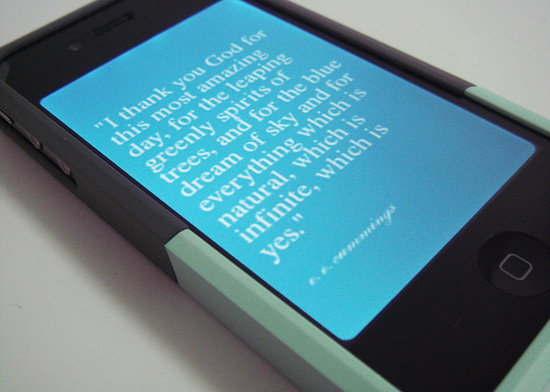This close-up photograph captures a smartphone, specifically an iPhone, positioned diagonally from the bottom right corner to the top left, against a white or off-white background. The phone’s display shows a quote in white text against a light blue background, reading, "I thank you God for this most amazing day, for the leaping greenly spirits of trees, and for the blue dream of sky, and for everything which is natural, which is infinite, which is yes," attributed to E.E. Cummings. The iPhone is encased in a protective cover that is silver and black in color. The device casts a shadow toward the lower left edge of the image, emphasizing its angular placement.